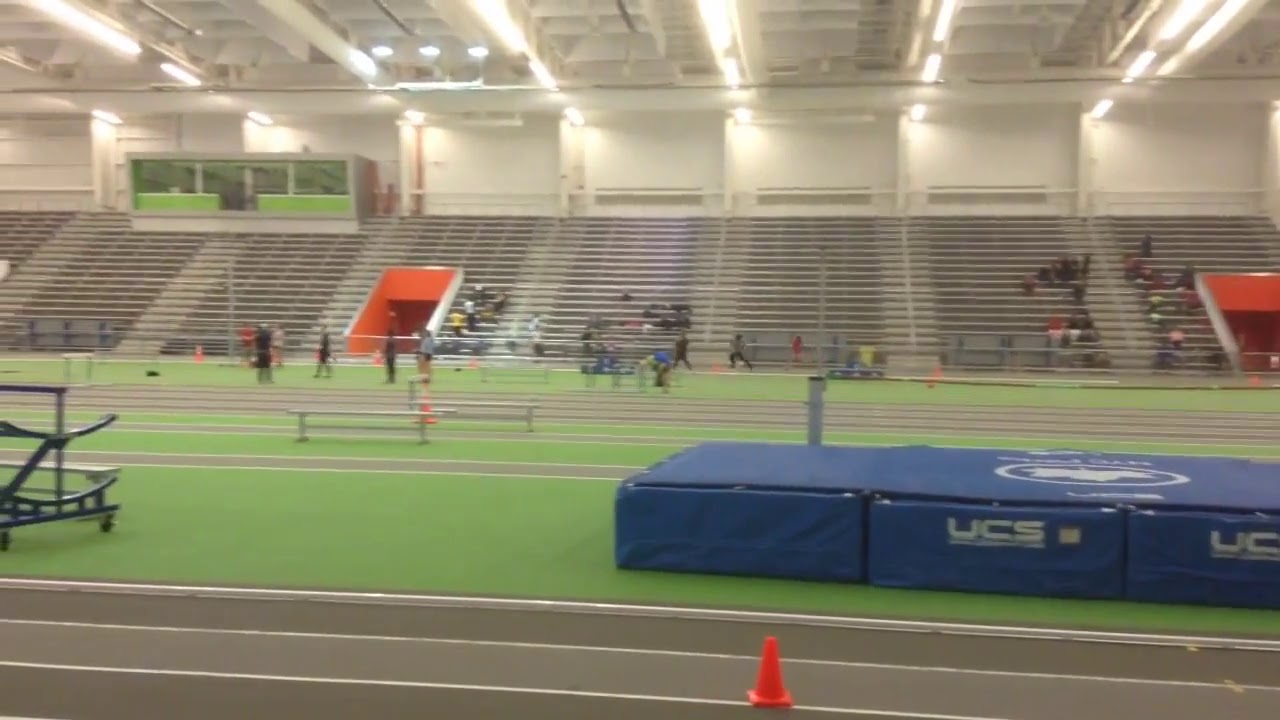This image captures the interior of a spacious indoor track and field stadium. In the foreground, a notable orange cone is situated on a gray track, leading the eye to a thick blue mat designed for gymnastics tumbles or landings. Surrounding the track, the inner field is scattered with various track and field equipment, including balancing bars and cones, amidst green patches, which appear to be an artificial surface rather than grass. In the background, bleachers with spectators are visible, some actively stretching, running, or simply watching the events. The structure of the stadium is highlighted by its exposed ceiling with large interior lights and an announcer's booth located towards the left wall. Orange tunnels underneath the bleachers suggest additional entrances or passageways. Overall, the image provides a detailed look at both the activity and infrastructure within a bustling indoor sports venue.